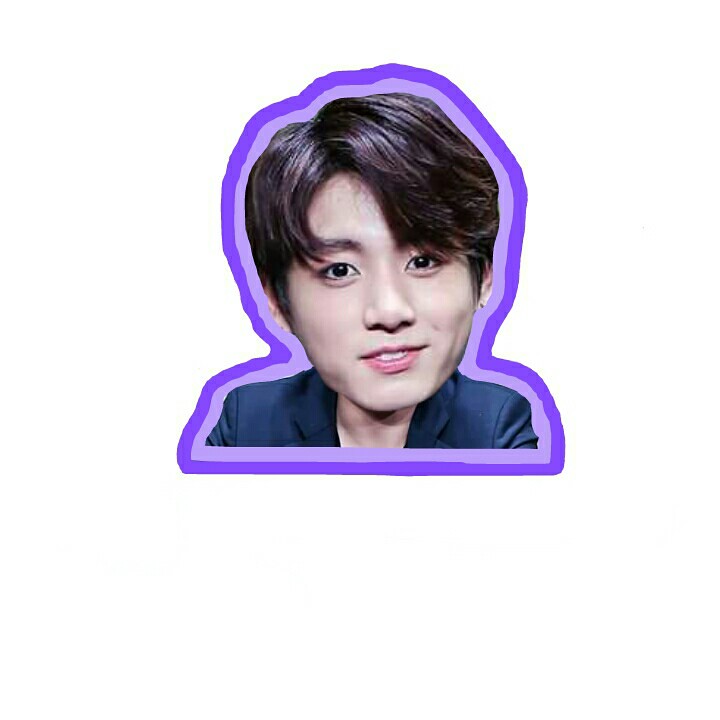The photograph is a detailed, edited image of a young Asian man, captured from the shoulders up. His hair is dark brown to black with subtle brown highlights, parted on the left side and styled in a short, fluffy manner with bangs gently resting over his dark brown eyebrows. He is dressed in an open-collared blue blazer and has a fair complexion. His face displays a slight smile, revealing his upper front teeth. Notably, the image has been edited to enlarge his head, giving it a bubble-head appearance. This unique portrait is artistically bordered first with a light lavender outline, and then further framed with a darker purple line, creating a sticker-like effect that emphasizes his head and shoulders.